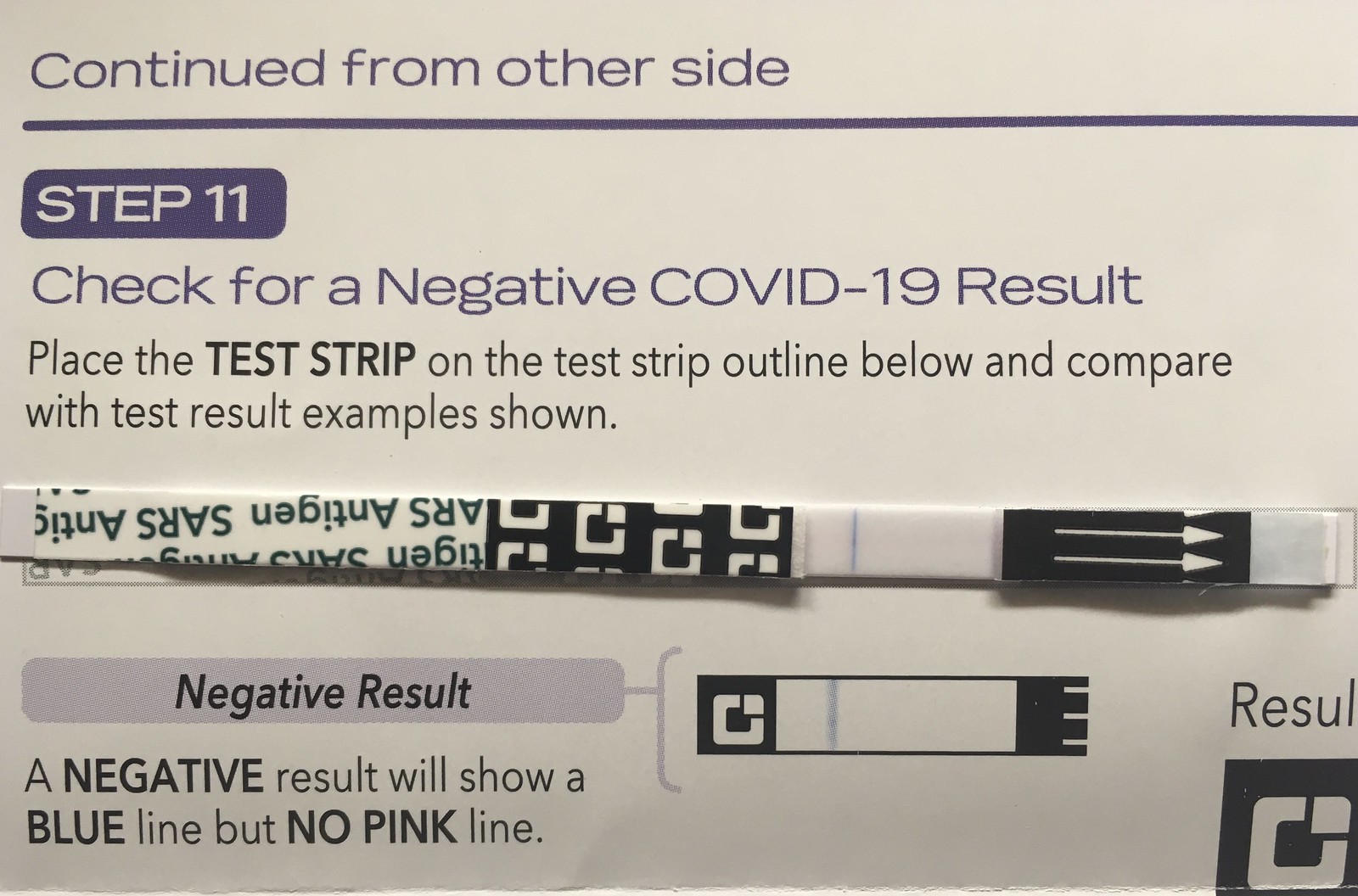The image displays an instruction sheet designed to help users interpret a COVID-19 negative result from a test strip. The sheet has a white background with black and light purple text, providing clear guidance. 

At the top of the sheet, in a purple rectangular box with white lettering, is "Step 11." Below this, a heading in purple reads, "Check for a negative COVID-19 result." The black text beneath the heading instructs users: "Place the test strip on the test strip outline below and compare with result example shown."

A test strip is placed exactly on the outlined area on the sheet, displaying a single blue line in the middle. According to the instructions, a blue line without a pink line indicates a negative result. The sheet includes a visual example of a negative result to further assist users in verifying their test outcome.

In summary, this image shows a comparison guide where users place their test strip on the provided outline to confirm a negative COVID-19 result, characterized by the presence of a blue line and the absence of a pink line.